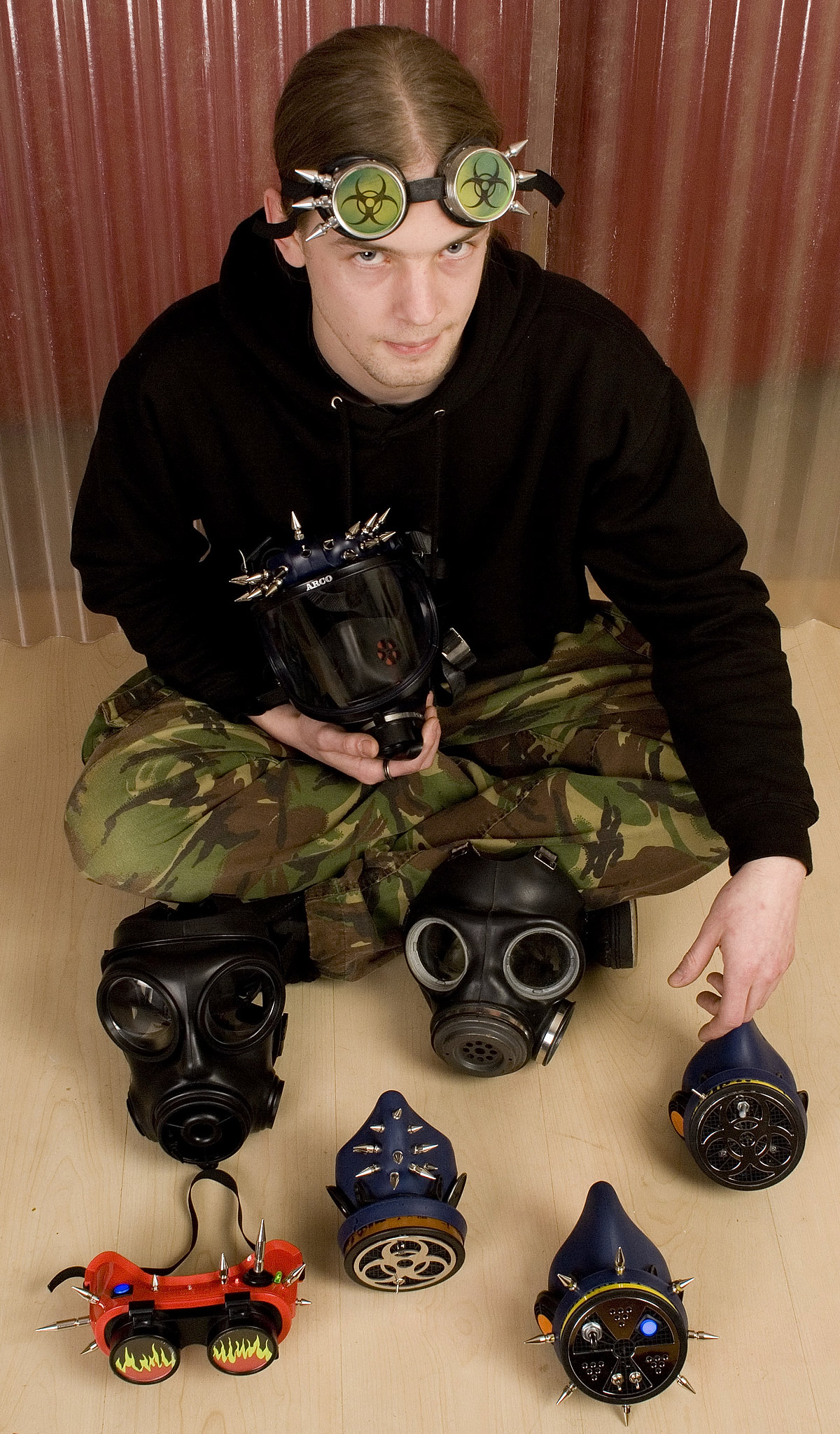In this photograph, a young man is seated cross-legged on a blonde hardwood floor. The background features a vertical corrugated silver metal sheet. He has fair skin, dark eyes, and long hair parted in the center, pulled back. He wears a black hoodie paired with jungle camouflage pants and black shoes. On his head, pushed up onto his forehead, rests a pair of round goggles with black symbols on a green background, accented by three chrome spikes on either side.

In front of him on the floor lie two black gas masks and an orange pair of goggles adorned with flame designs over the lenses. Additionally, there are three different filter attachments festooned with an assortment of chrome spikes and symbols, some bearing the nuclear symbol. The man is holding one of the black gas masks in his hand and gazes up at the photographer, creating a striking, post-apocalyptic vibe.